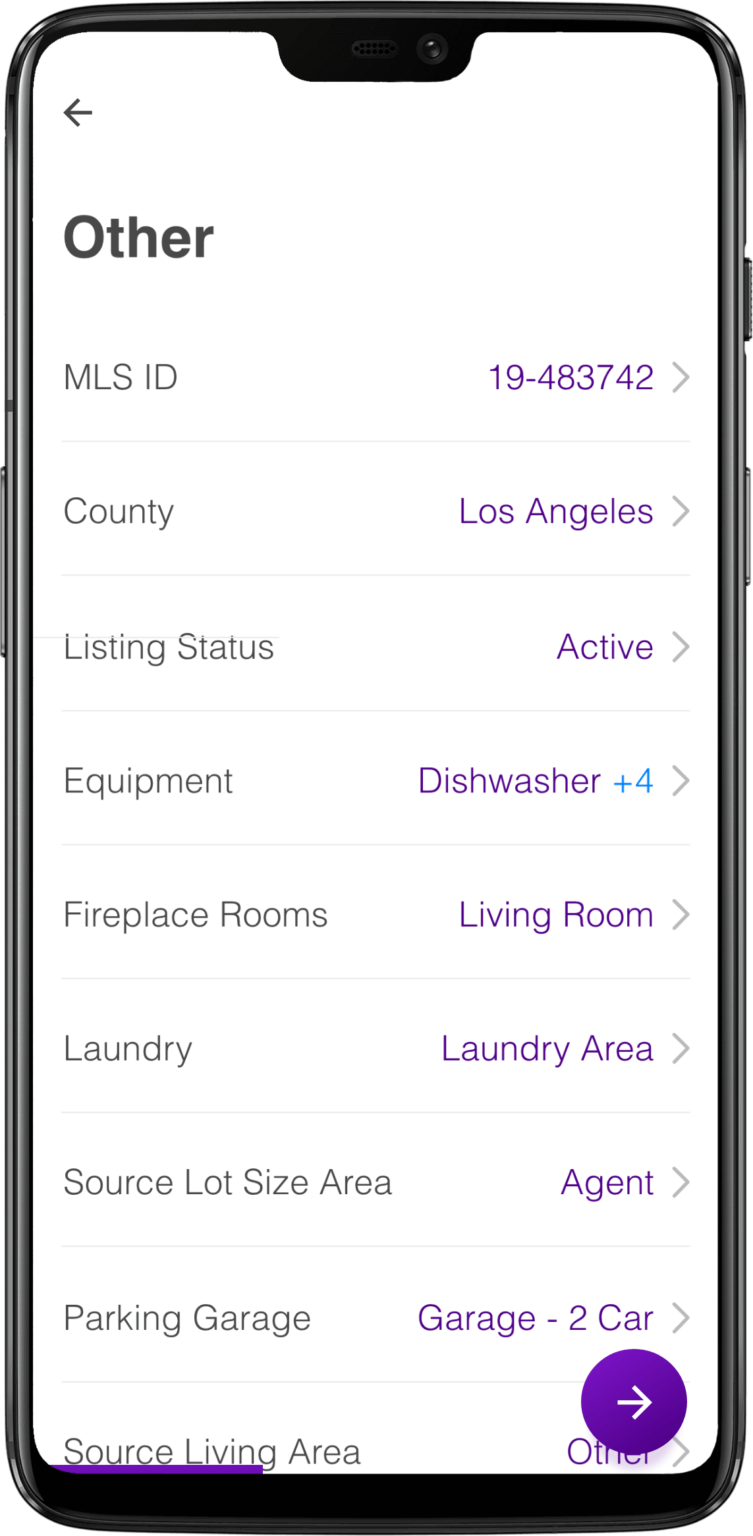The image is a detailed screenshot of an app's customization tab, designed to showcase specific features and details related to listings. The full phone screen is displayed prominently, likely for the purpose of advertising the app or highlighting this particular section. 

In the upper left corner, 'Other' is displayed in dark gray. Below, a series of customizable fields are listed. These fields include:

1. MLS ID
2. County
3. Listing Status
4. Equipment
5. Fireplace Rooms
6. Laundry
7. Source Lot Size Area
8. Parking Garage
9. Source Living Area

On the right side, corresponding field entries are displayed in purple and blue:

1. 19-483742
2. Los Angeles
3. Active
4. Dishwasher
5. Plus four (in blue)
6. Living Room
7. Laundry Area
8. Agent
9. Garage - Two car
10. Other

This detailed breakdown presents the various attributes and specifications relevant to a property listing, offering an in-depth look at the customization options available within the app.